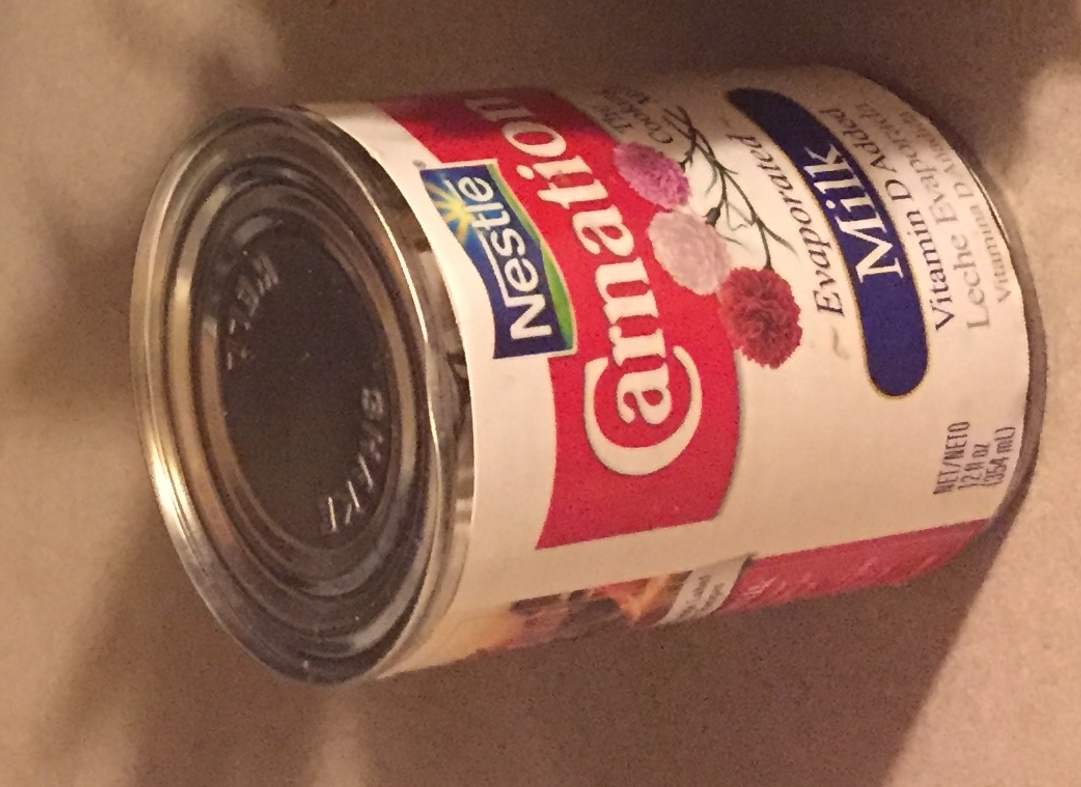The photograph showcases a brightly lit indoor setting featuring a medium-brown surface. Resting on this surface is a steel can of Carnation Evaporated Milk, prominently positioned in a well-illuminated environment that casts distinct shadows. The front of the can's label predominantly showcases a white background adorned with several colorful elements. Near the top, a blue banner boldly displays the word "Nestlé" in white lettering, complemented by stylized yellow sun rays radiating from it. Below this, another banner in vivid red reads "Carnation." Adding a touch of elegance, three illustrated Carnation flowers are depicted beneath this banner: one pink, one in a creamy off-white hue, and one red. The partial view of the back label reveals another red section, and it seems to feature an image of a dish that can be prepared using the evaporated milk, though the details of this dish remain unclear from the current angle.